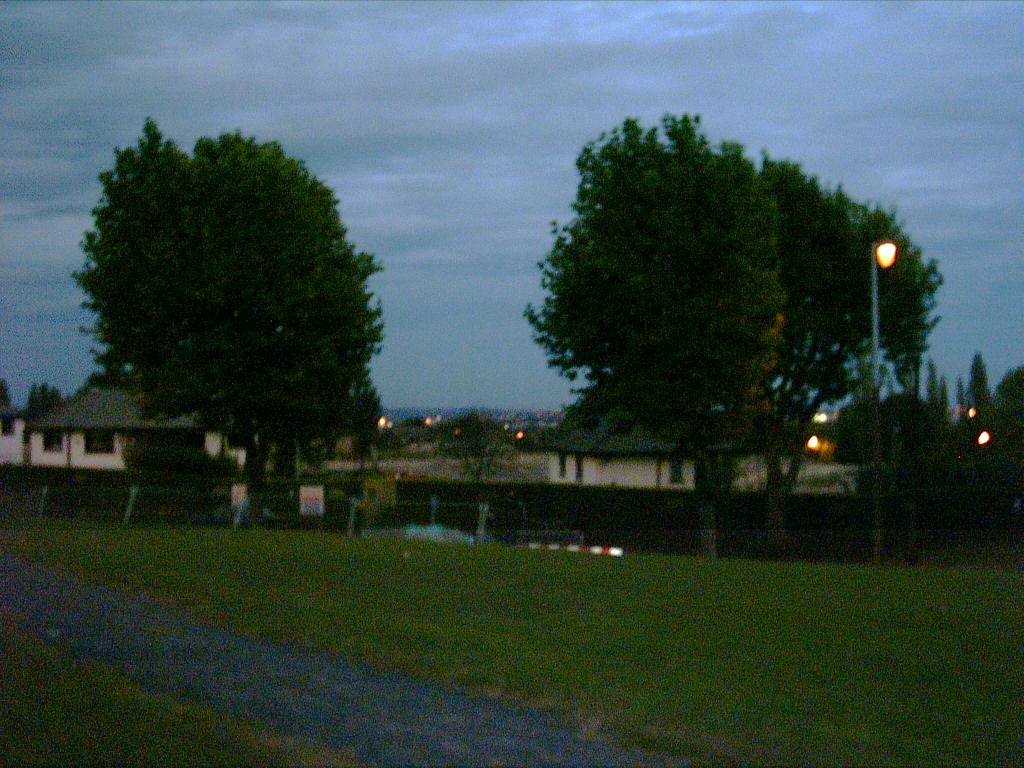This photo, taken in the late evening as the sun sets, captures a serene neighborhood scene under a cloudy, dusky-blue sky. At the forefront is a green grassy area, intersected by a diagonally cut gravel path of dark gray pebbles. This path extends from the center to the lower left corner of the image. Flanking the scene are three large, full trees—one robust and circular on the left, and two more spread out, including one visible on the right near a street lamp. Beyond the trees, a fence stretches across the entire photo, a blend of chain-link and stockade styles.

Behind the fence stand two cream-colored houses with dark roofs, nestled under the trees. The house on the left features a typical rectangular roof, while the one on the right boasts a design with an upward curling end, reflecting its unique circular section. Lights illuminate the area, including streetlights visible in the background, hinting at a broader neighborhood. Scattered in the vicinity are various objects, including a small red and white striped item lying horizontally on the ground. This picturesque setting appears to be viewed from a walking trail, capturing the tranquil ambiance of the approaching night.